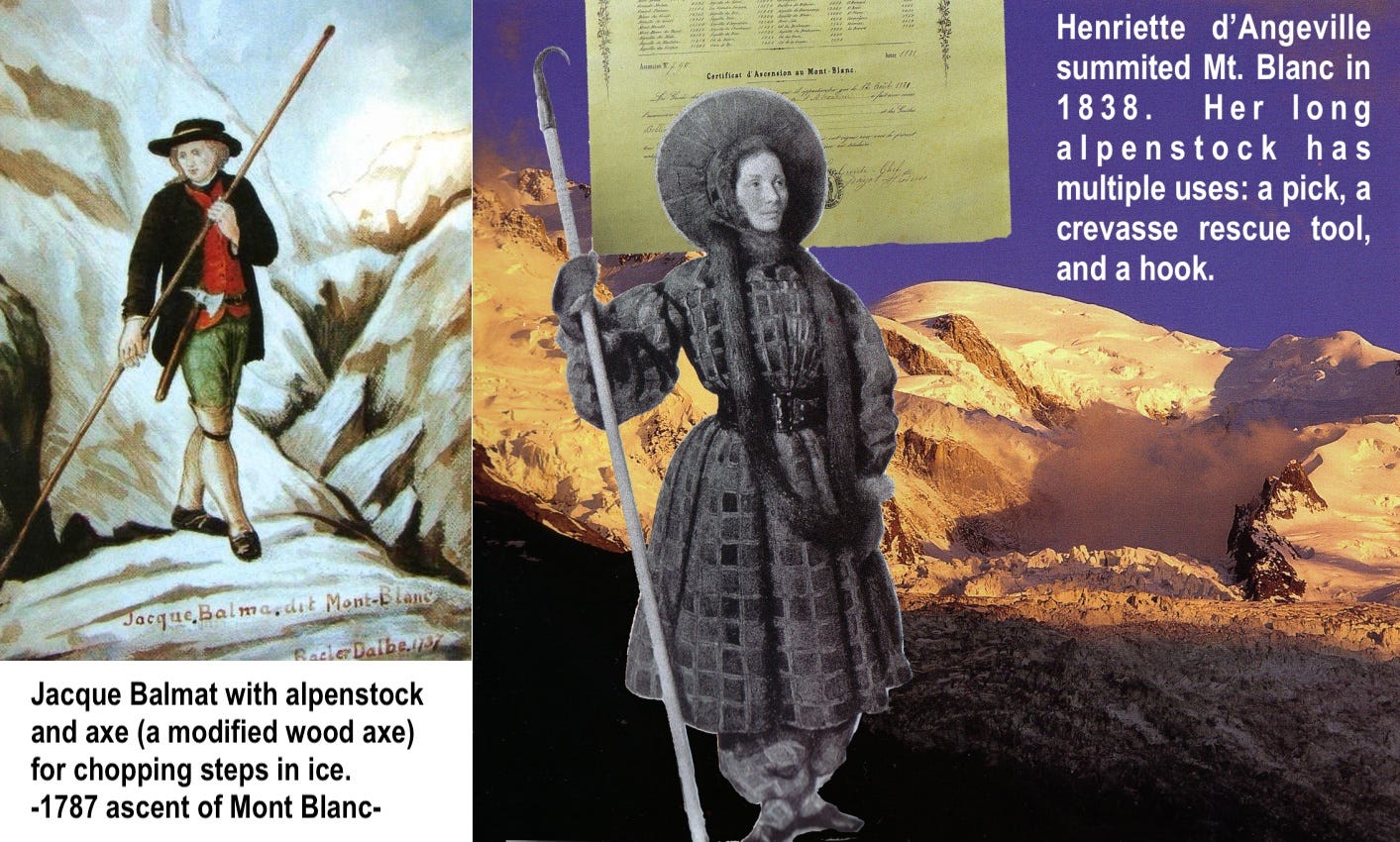The illustration consists of two historical images seemingly taken from a history book, depicting notable climbers of Mont Blanc. On the left, there is a man, Jacques Balmet, dressed in a colonial-style outfit featuring a brown coat over a red shirt, green knee-length shorts, white knee-high socks, and brown shoes. He holds a long pole and an axe, identified as an "Alpenstock and Axe, a modified wood axe for chopping steps in ice," associated with his 1787 ascent of Mont Blanc. Balmet stands on a rugged terrain of boulder-like blocks, suggesting a challenging climb.

The right image depicts Henrietta D’Angeville, who ascended Mont Blanc in 1838. She is dressed in a two-tone black and gray coat that extends below her knees, along with pants and a large brimmed hat adorned with a long scarf. She holds an Alpenstock, a multifunctional tool used for picking, rescuing from crevices, and hooking. Behind her lies a rocky, mountainous backdrop, and there appears to be some manuscript-like text, though it's not legible. The background blends into a purple-hued sky, enhancing the dramatic and adventurous atmosphere of the scene.